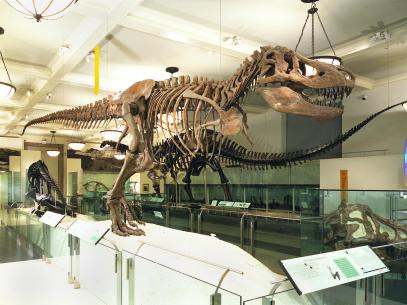This photograph captures a detailed and immersive view of a dinosaur fossil exhibit at a natural history museum. Dominating the foreground is a fully intact skeleton of a Tyrannosaurus rex, positioned on a glass stand with lights illuminating it from below. The T-Rex skeleton faces towards the right side of the image, its imposing structure complemented by a placard on a glass railing nearby, though the text is not legible. 

In the background, adding depth and contrast to the scene, is another prominent dinosaur skeleton with a long neck and tail, likely that of a Brontosaurus or Brachiosaurus. This secondary skeleton faces the opposite direction, towards the left side of the image. The high ceiling above features several large globe lights that enhance the visibility and ambiance of the exhibit. The surrounding area includes additional glass cases which potentially hold smaller fossils and artifacts, contributing to the comprehensive display that is characteristic of a museum setting. 

The overall arrangement and the familiar setting hint that this exhibit might be part of a well-known collection, possibly one that visitors might recognize from previous trips to the Natural History Museum.